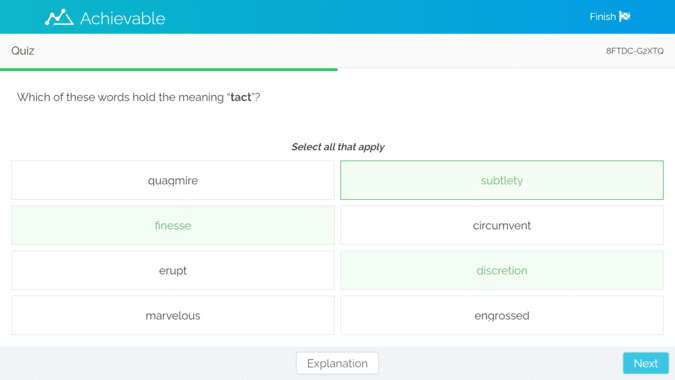The image predominantly features a blue band across the top. On the left side of this band, the word "Achievable" is displayed, suggesting an aspect of goal setting or achievement. On the right side, the word "Finish" appears alongside a finish flag icon, indicating the completion point. Below this blue band, the word "Quiz" is prominently displayed.

A green instructional line beneath the band reads, "Which of these words holds the meaning 'tact'? Select all that apply." The options presented are: "quagmire," "finesse," "erupt," "subtlety," "circumvent," "discretion," and "gross." The words "finesse," "subtlety," and "discretion" have been selected, turning a light green to signify correct choices.

At the bottom center of the image, a white button with black or gray text reads "Expand." To the right of this, a turquoise button labeled "Next" is visible.

The image appears to depict a practice question from a study program, specifically for the MBLEX exam (Massage and Bodywork Licensing Examination) in the United States, providing a realistic example of practice questions used to prepare for the exam.